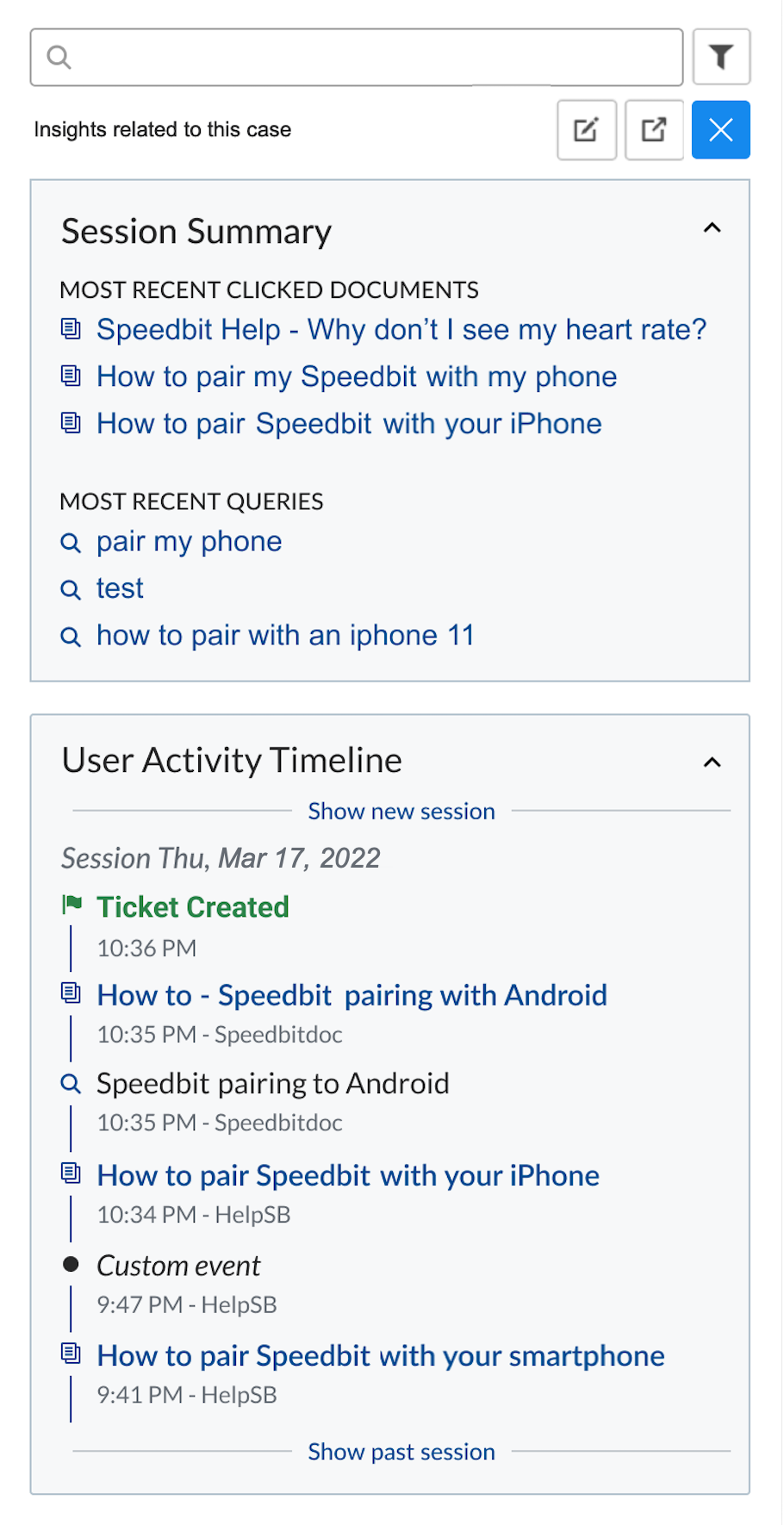**Screenshot Description:**

The screenshot captures a user interface likely from a software application that provides detailed insights related to a specific case. The layout is organized into two distinct sections: "Session Summary" and "User Activity Timeline."

**Top Section:**

- **Search Bar**: Located at the top of the screenshot for ease of access.
- **Title**: Bold black text reads "Insights Related to This Case."
- **Icons**: Next to the title are various icons enclosed within squares.
- **Cancel Button**: A blue square marked with an 'X,' allowing users to cancel the current view.

**Session Summary:**

- **Subheading**: "MOST RECENT CLICKED DOCUMENTS" in all capital letters, emphasizing the section for recent interactions.
- **Items Listed**:
  - "Speech Help"
  - "How to pair my Speed bit with my phone"
  - "How to pair a Speed bit with your phone"
- **Most Recent Queries**:
  - Represented with blue-colored magnifying glass icons next to them:
    - "Pair my phone"
    - "Test"
    - "How to pair with an iPhone 11"

**User Activity Timeline:**

- **Subheading**: "User Activity Timeline" presented as a horizontal bar.
- **Details**: Highlights activities segmented by time, focusing on a session from Thursday, March 17, 2022:
  - **Session Start**: "Ticket created at 10:36 PM."
  - **Activities**: Sequential list of actions taken at specific times:
    - "How to pair bit pairing with Android at 10:35 PM."
    - "Speed bit pairing to Android at 10:35 PM."
    - "How to pair Speed bit with your iPhone."
    - "Custom Event and How to pair Speed bit with your smartphone."

This comprehensive caption summarizes the contents and layout of the screenshot, emphasizing the structure and specific details of the user interactions shown.